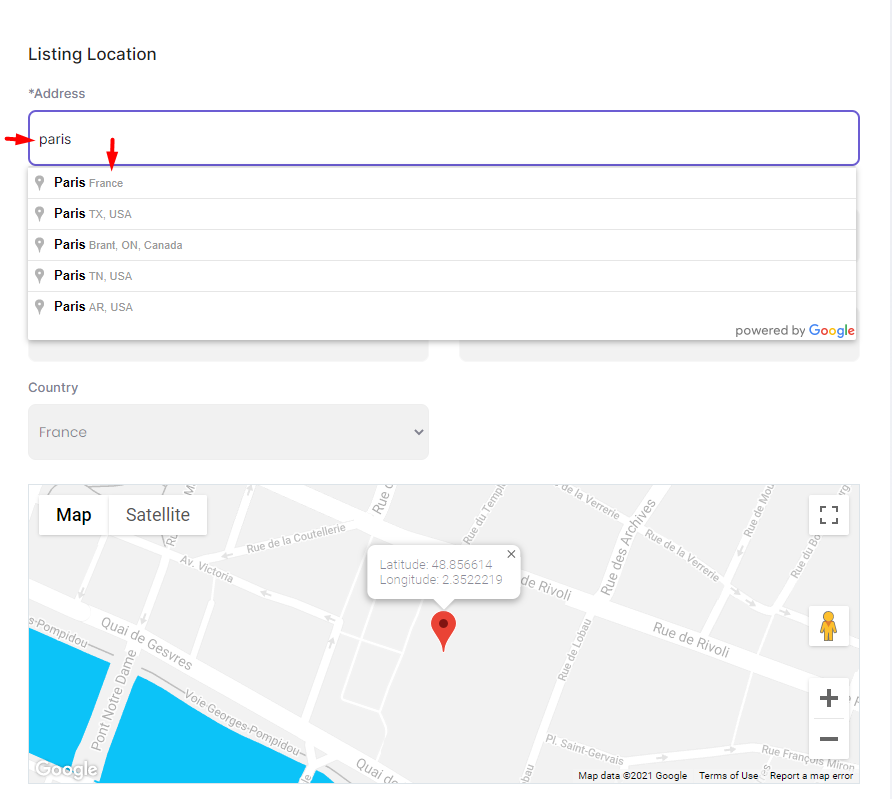This image is a detailed capture of a website interface centered around geographic location listings. The background is white with a black header displaying the text "Listing Location." The address field is highlighted with a blue box and marked with an asterisk, indicating a required input. 

A red arrow points to the text "Paris" in black, while another red arrow directs attention downward to a list of various cities named Paris, including:
1. Paris, France
2. Paris, Texas, USA
3. Paris, Brant, Ontario, Canada
4. Paris, Tennessee, USA
5. Paris, Arkansas, USA

At the bottom, the phrase "Powered by Google" is accompanied by the Google logo in its recognizable blue, red, gold, and green colors. Directly below this, there is a dropdown box labeled "Country France," followed by a Google Maps view featuring a 2021 copyright date.

The Google Maps view includes options for "Terms of Use" and "Report a Map Error." Two selectable boxes appear here — “Map” and “Satellite” — with the “Map” option currently selected. The map view itself depicts Paris with visible streets and notable landmarks. A white pop-up box shows latitude and longitude coordinates: 48.856614 (latitude) and 2.3522219 (longitude), marked by a prominent red location pin.

Additional interface elements include a white box with a black square, a white box featuring a gold person icon (likely for Street View), a white plus sign, and a white and gray minus sign, presumably for zooming in and out on the map.